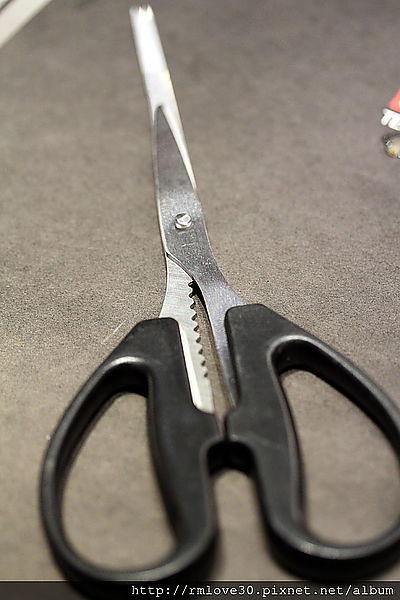This is a detailed, close-up vertical photograph of a pair of scissors, prominently positioned from the bottom left to the top right corner of the image. The black plastic handles, with their smooth oval shapes, are situated at the bottom right, near the center of the image. The stainless steel blades extend diagonally, pointing toward the top left. The scissors are placed on a gray surface that might be a table, with a white piece of paper beneath them. The image has a black bar at the bottom with white text that reads "http://rmlove30.pixnet.net/album." Additionally, a subtle red element is visible at the top right, while a white object appears faintly in the top left corner. The light reflects off the scissors, making the tips appear almost white due to the high gloss on the metal.